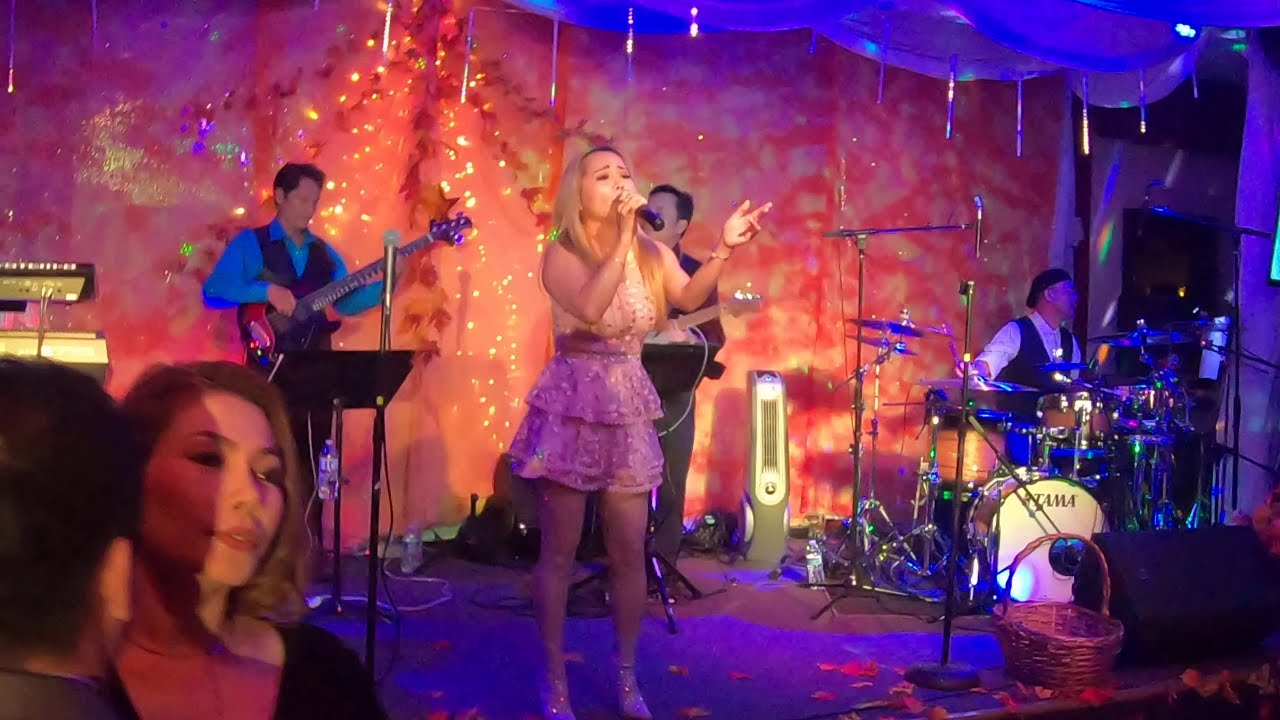The photograph captures a vibrant indoor stage performance featuring a blonde singer in a shimmering, short pink dress and matching heels. She stands center stage, energetically singing into a microphone held close to her mouth while gesturing with her free hand. Her dress, detailed with layers, offers a twirly, feminine aesthetic. Behind her, the stage is adorned with sparkly orange and blue-purple backdrops, enhanced by bright, indoor lighting. To her right sits an older drummer wearing a white shirt, dark vest, and a black hat, intently engaged in the rhythm. On her left, a guitarist dressed in a long-sleeved blue collared shirt and black vest plays energetically. Another guitarist, partially obscured by the singer, also contributes to the musical harmony. In the lower left corner, a couple is seen dancing, adding an extra layer of liveliness to the scene. Scattered rose petals on the blue-lit stage enhance the visual charm of the performance.